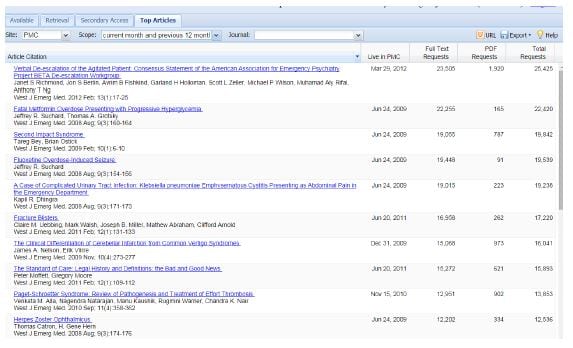A nostalgic webpage design, possibly from the early 2000s, is captured in this image. The page features a header in a light blue shade, reminiscent of the Windows XP era, with bubble-shaped tabs that lend a vintage charm. The tabs, from left to right, include one partially obscured, followed by "Retrieval," "Secondary Access," and "Top Articles." The "Top Articles" tab is prominently selected, indicated by its bold, black font and lighter background.

Below the tabs, a drop-down menu is present. On the left, a label reads "Site" with the option "PMC" selected in the dropdown. Adjacent to it, the "Scope" is defined with another dropdown displaying "Current Month in Previous 12 Month," though the text is cut off at the "H." Further down, a "Journal" dropdown showcases a blank white space, indicating no current selection.

To the right of these dropdowns are three options: "URL," "Export," and "Help." Enhancing the vintage design, a header area fades from light blue at the bottom to white at the top, creating a subtle 3D effect. In bold black text on the left, "Article Citation" is displayed, followed by tabs titled "Live in PMC," "Full Text Requests," "PDF Requests," and "Total Requests."

Beneath these tabs, a series of clickable URLs are listed, identified by their dark blue, underlined text. Each URL is followed by detailed information in black text, including various dates and numerical data, neatly organized in columns under the respective headings. This meticulous layout encapsulates the functional yet charmingly dated aesthetic of early 21st-century web design.